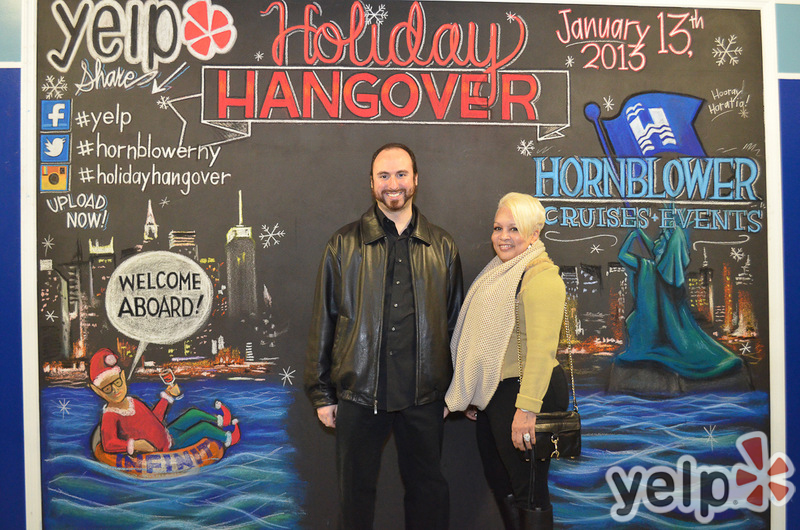In this detailed image, a man and a woman pose in front of a vibrant, gray mural that prominently features the words "Holiday Hangover" in the center in light red text. Additionally, "January 13, 2013" is inscribed to the right of this central text. The mural also depicts a lively city scene with a river in the foreground, where an elf floats with a speech bubble that reads, "Welcome Aboard." The man, standing in the center, wears a shiny black leather jacket over a black button-up shirt, paired with black pants. He has dark hair, a beard, and a mustache, and he flashes a smile for the camera. To his side, the woman stands in profile, facing him. She has striking platinum blonde hair and is dressed in a yellowish-beige long-sleeved shirt, a beige scarf, black pants, and carries a black purse. The iconic Yelp logo is positioned in both the top left and bottom right corners of the picture.